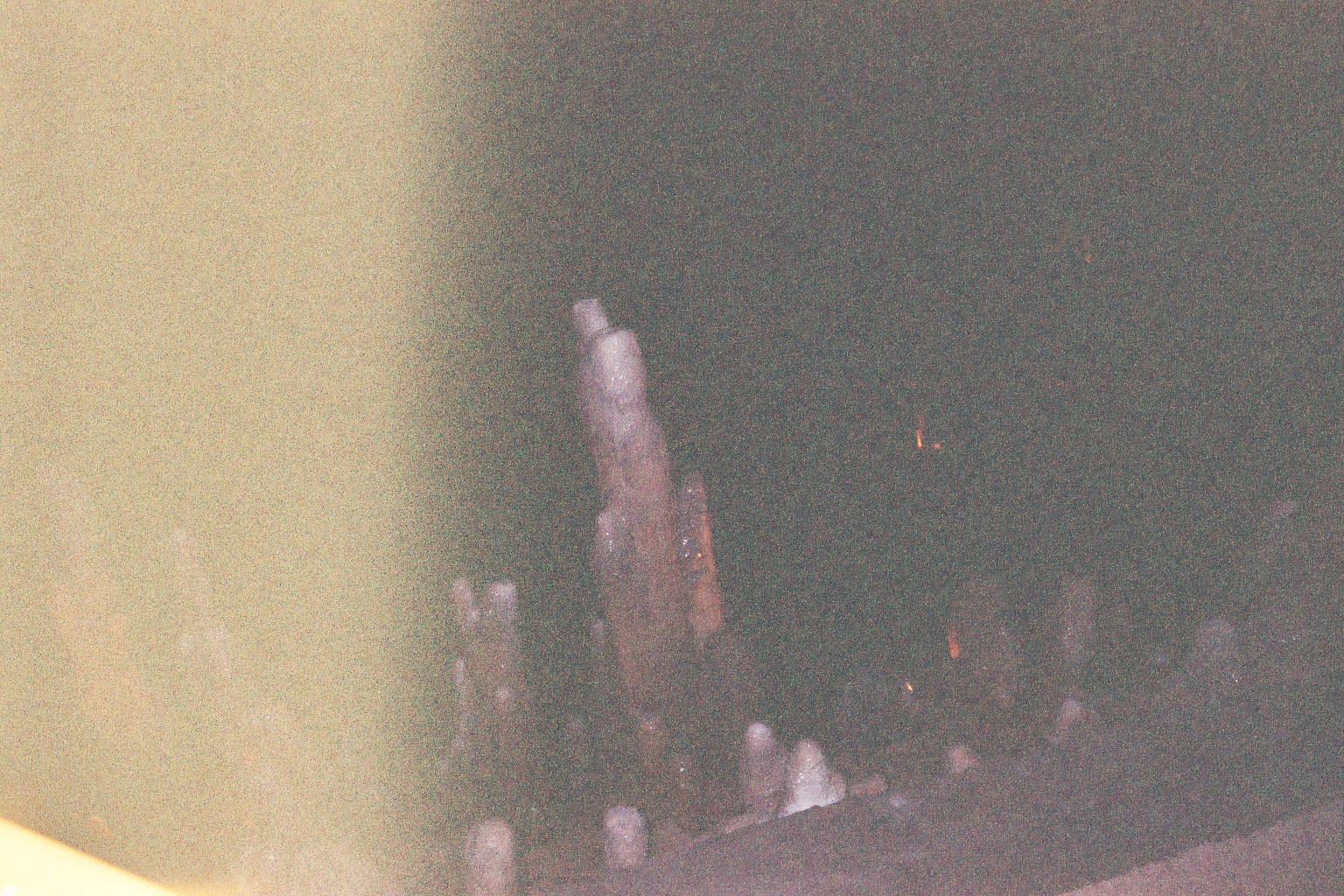An awe-inspiring view from inside a cavern reveals a mesmerizing landscape of eerie rock formations. Stalactites hang like ancient chandeliers from the high ceiling, their damp surfaces shimmering in the faint light, while stalagmites rise from the cavern floor, their jagged tips reaching upward as if in silent conversation. The formations boast a palette of muted colors, ranging from earthen browns to hints of green and blue, reminiscent of wet paint. The dimly lit cavern, shrouded in shadows, exudes an otherworldly, almost spooky atmosphere that amplifies the sense of exploration and discovery.